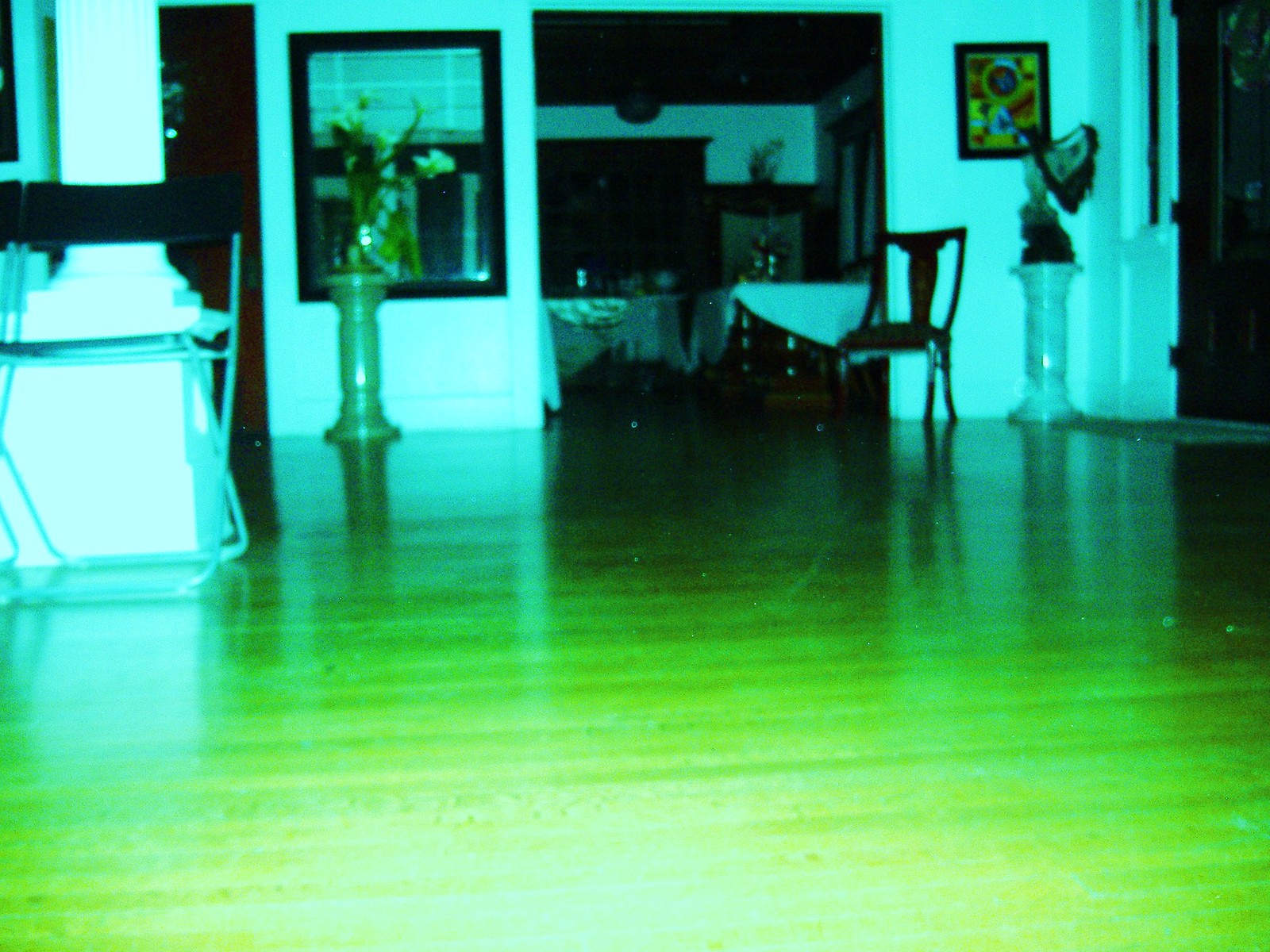This color photo, though distorted by harsh neon green lighting that oddly illuminates the brown hardwood floor, offers a glimpse into a somewhat cluttered yet quaint interior. The bottom part of the image is dominated by this unnatural green light, making the wooden floor appear almost glow-in-the-dark. On the right-hand side, there is a wood table partially visible, while a white chair with a black back rests nearby, suggesting a formal dining setting.

In the distance, a tall vase containing tallow is perched on a stand, flanking an open doorway that appears to lead into a dining room. The walls are a stark white, and to the top right, a painting with black, yellow, red, and blue designs and circles can be seen. Opposite, on the top left, a window with drawn-up blinds allows some light to spill in.

Adjacent to this window, another tall stand similar to the one with the vase supports another floral arrangement. Next to the open doorway, a glimpse of a black door frames the far right-hand side. Passing through the doorway reveals a dark wooden dining table draped with a white cloth, surrounded by chairs. Dominating the back wall of this adjacent room is a large black china cabinet, featuring multiple little windows, housing various items that hint at the room's full, lived-in aesthetic.